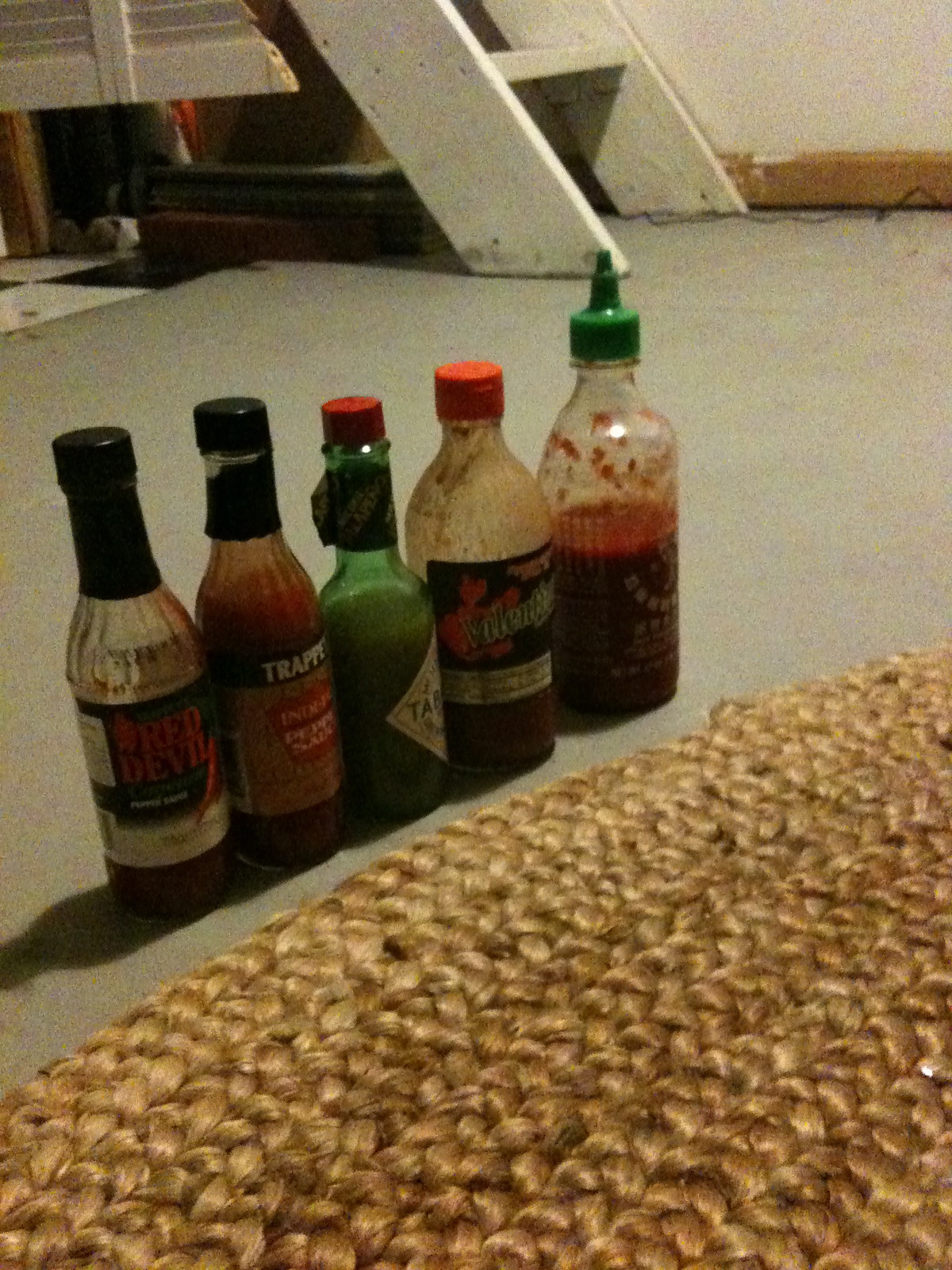This photograph depicts a collection of five hot sauce bottles arranged diagonally in a row on a variegated brown woven mat placed on a gray cement floor. The image shows various brands and types of hot sauces, most of which are at least halfway used. From left to right, the lineup includes: Red Devil pepper sauce with the least amount remaining, a bottle labeled Trappers with a black cap, the original green-capped Tabasco, a bottle that appears to read Villain with a red cap, and a more than half-empty green-capped bottle of Sriracha. A shadow cast by a light source on the right edge emphasizes the bottles’ placement. In the background, there's a white wooden ladder leading either to an attic or a basement, placed against a cement wall, suggesting this setup is in a basement.